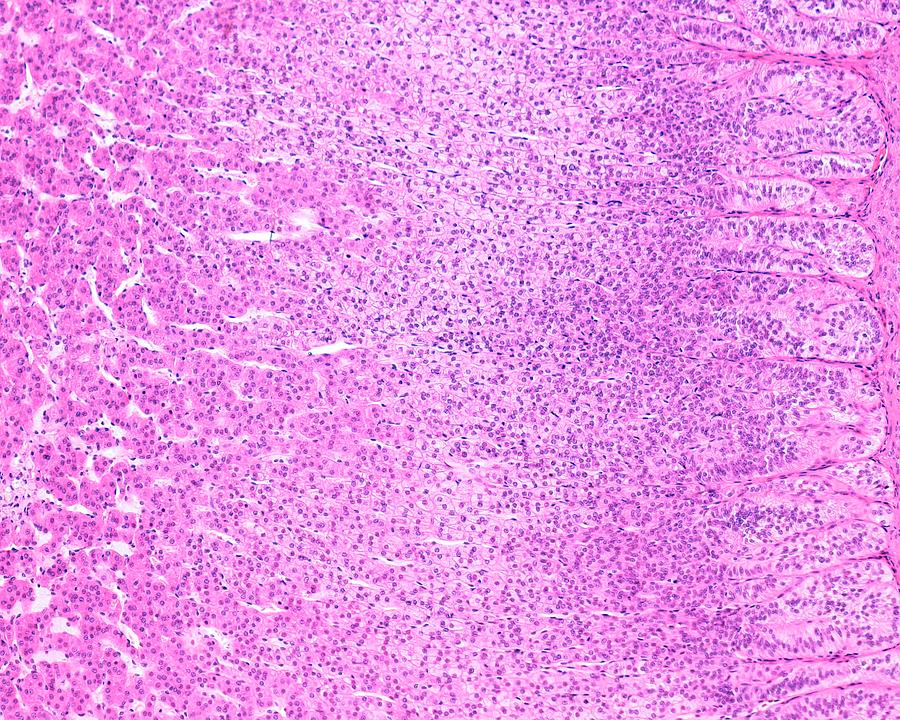The image appears to be a high-magnification microscopic view resembling a tissue or cell slice dominated by a vibrant pinkish-purple hue with intricate details. The central focus is an area with a lighter background, filled with numerous tiny purple dots scattered throughout, some clustered and others spaced apart. On the left side, there are noticeable white stains, horizontal marks that snake across, adding to the textured appearance. In contrast, the right side features bulbous, almost finger-like shapes that stand out amidst the darker pink markings. The entire composition is rich with snaking white lines and dots that create a visually complex and highly detailed scene.